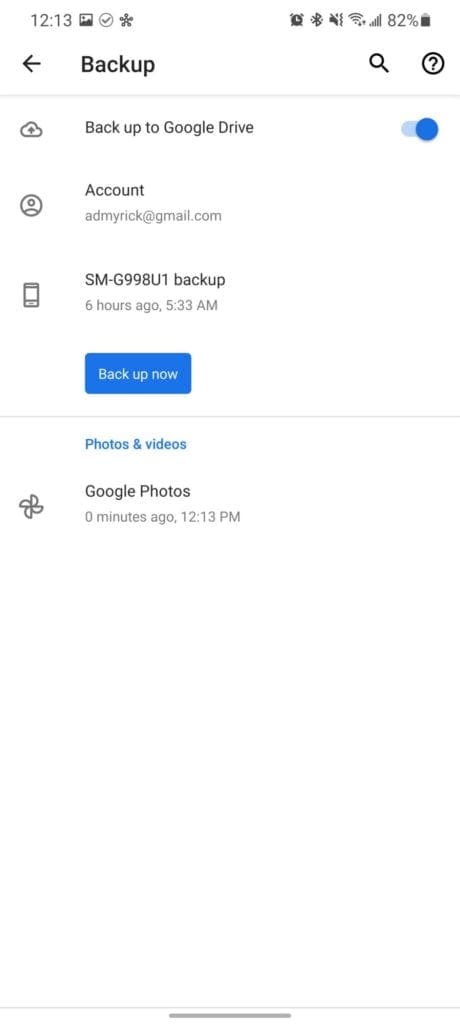Screenshot Description:

The image depicts a screenshot of a website accessed on a mobile phone. At the very top, the status bar shows the time as 12:13 PM, followed by a series of icons: a photo symbol, a circle with a check mark, and a flower symbol. On the right side of the status bar, there are additional icons including an alarm clock, an unknown symbol, a notification bell with a slash through it (indicating notifications are muted), a Wi-Fi signal with full strength, a 5-bar signal indicator, and a battery icon displaying 82% charge.

Below the status bar is a navigation bar with a left-facing arrow labeled "Backup" on the left side, and a magnifying glass (search) icon and a circle with a question mark (help) icon on the right side.

The main content area features a cloud image accompanied by the text "Backup to Google Drive." Below this is an on/off switch which is toggled to the "on" position. Underneath the switch, there is a profile picture symbol next to the account information "admyrick@gmail.com."

Further down, there is an image of a cell phone labeled "SM-G998U1 backup," indicating the last backup occurred 6 hours ago at 5:33 AM. Next to this information, there is a blue button labeled "Backup now."

Below this button, there is a clickable link in blue text that says "Photos and videos." At the bottom of the screenshot, there is a fan symbol next to the text "Google Photos," showing that the last sync occurred 0 minutes ago at 12:13 PM.